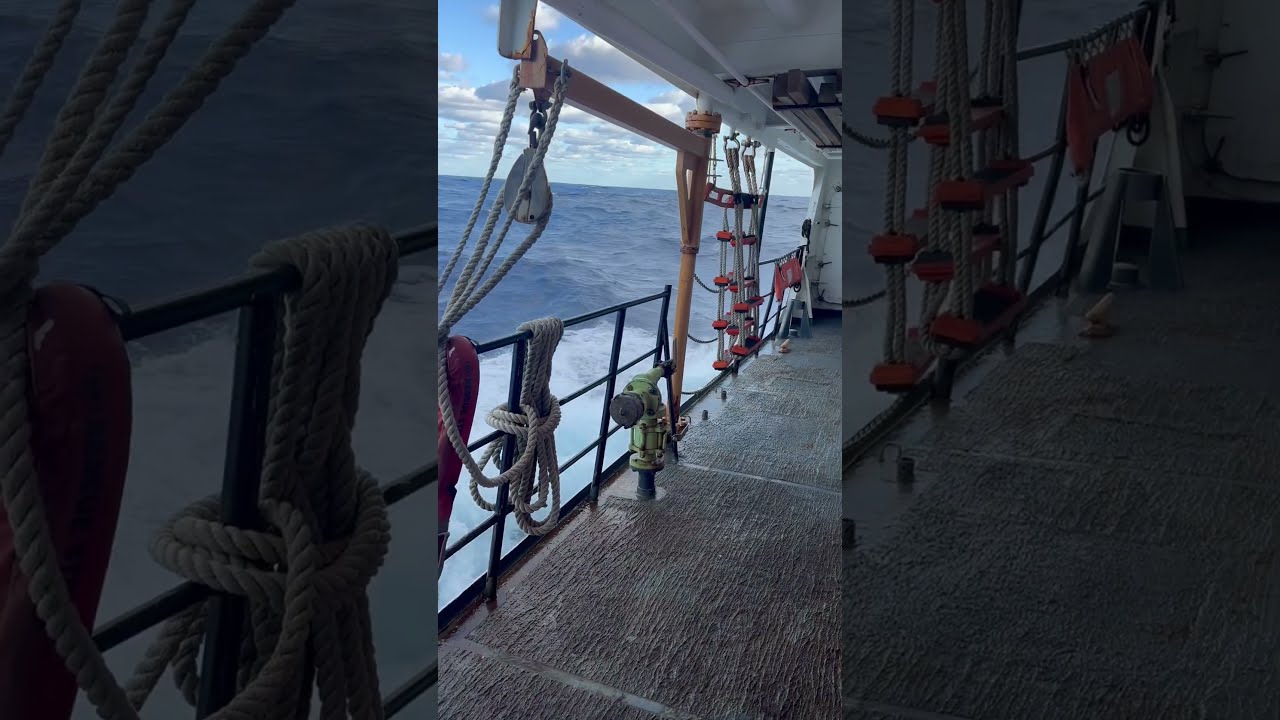The image depicts a detailed scene on the side of a commercial vessel, either a fishing boat or a freight boat, captured from a first-person perspective. The deck is rugged with a textured brown floor and a distinct charcoal ground. There's a greenish pipe centrally visible. Surrounding the deck, one can see various maritime equipment including sturdy guard railings, large ropes, pulleys, cranes, and a red ladder-like structure. Both red and gray ropes are tied in seamen’s knots and ready to be thrown overboard. The boat is in the middle of the ocean, which appears turbulent with white bubbles on top of the waves. The sky is a mix of blue and white-gray clouds, hinting at rough sea conditions. The image also features a white roof and tan, green, blue, white, and orange color elements. No people are visible in this section, and it appears to be a still shot, possibly a screen grab from a video.